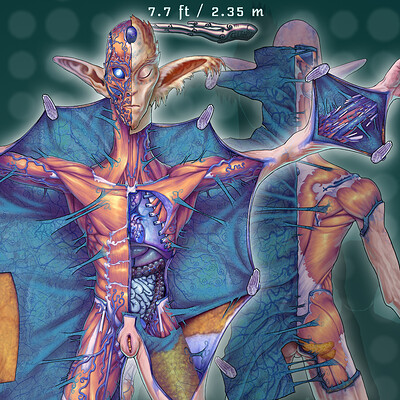The image is a digitally generated, highly detailed anatomical drawing of a humanoid fantasy alien creature. The creature stands in a spread-legged, arms-open-wide pose against a dark green background with lighter green circles scattered across it. At the top of the image, a label reads "7.7 FT / 2.35 M" in white text.

The alien's head is elongated with a tall forehead, a pointed chin, and unusually long ears reminiscent of Yoda, covered with short fur, extending outward. The creature's skin, bluish in color and marked with darker blue blood vessels, is peeled back and held by retractors, revealing a spectrum of internal structures.

Beneath the flayed skin, the exposed musculature appears in shades of orangish-pink. Portions of the muscle tissue, especially on the right side of the abdomen, have been cut away to uncover the alien’s internal organs displayed in various colors: the digestive tract and other organs appear in shades of blue and black. The intricate display includes details of the respiratory system, nerves shown in red, and portions of the brain and skull, all highlighted in distinct colors. In addition, the image features a rear view of the creature showcasing its musculature.

The attention to anatomical details, including sections of the digestive, respiratory, and nervous systems, implies a blend of artistic creativity with scientific-like precision, emphasizing a thorough dissection. The addition of light blue wings behind the figure adds to its otherworldly appearance, contributing to its fantastical and alien nature.